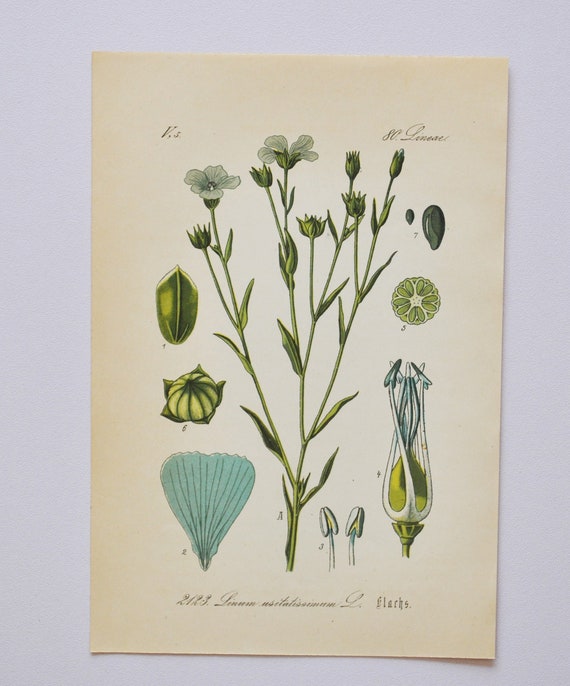The image appears to be an intricately detailed artwork or illustration, likely from a book, depicting the various stages of a flower's development. Set against a background resembling old, slightly brown paper, it features seven distinct images arranged in sequence. The main illustration in the center showcases a green stem that branches into multiple smaller stems, each culminating in buds and blooming flowers with delicate white petals. Surrounding this central illustration are additional images that appear to chronicle the flower's life cycle from seed to bloom. On the left side is an image of a green seed in the early stages of germination, progressing to a half-opened bud and eventually to a blue flower. On the right side, there is a depiction reminiscent of a lime slice with intricate white lines on the exterior transitioning to blue within, bearing a round shape with small leaves or petals around a central seed. The artwork includes cursive text at the top left, top right, and bottom, but the writing is faint and difficult to read. The entire image rests on a white surface, perhaps a table. The main colors in the illustration are the soft browns of the paper, the vivid greens of the stems and buds, and the blues and whites of the flowers and petals.